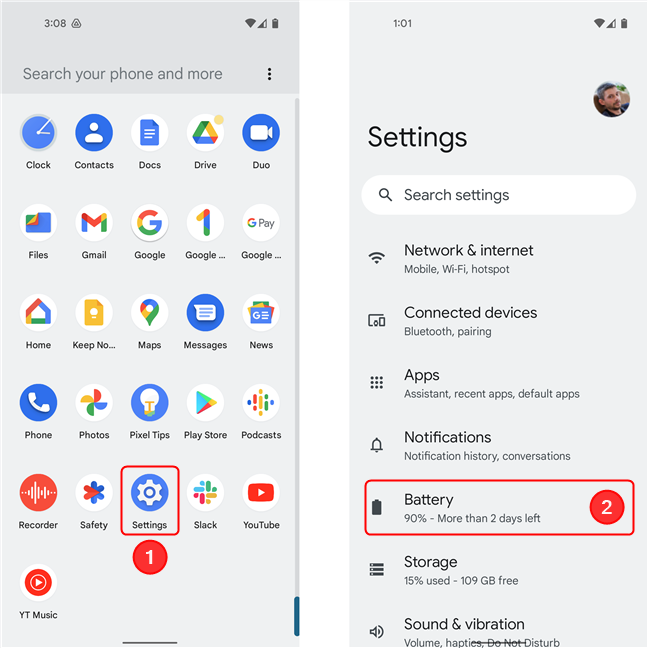The image features two adjacent cell phone screens, likely used for educational purposes. 

On the left screen, the time is displayed as 3:08 PM in the top left corner. To the right are indicators for cellular signal, Wi-Fi, and battery status. The screen displays a search bar labeled "Search your phone and more," and showcases numerous icons. Notably, a settings icon located at the bottom has a red box around it and a red circle with the number one inside, indicating a notification or update.

The right screen shows an in-depth view of the settings menu. The header reads "Settings," and one of the highlighted options is "Battery," which shows a status of 90% with more than two days of battery life left. This option also has a red box around it, accompanied by a red circle with the number two. The list features several other settings options, each with differing colors such as red, blue, white, yellow, green, gray, black, and orange.

Additionally, there is a profile picture of a Caucasian man with dark hair, a mustache, and a beard. It seems the image serves as a step-by-step guide, leading the user through the phone settings to monitor battery usage. There are no further instructions provided on what the next steps might be.